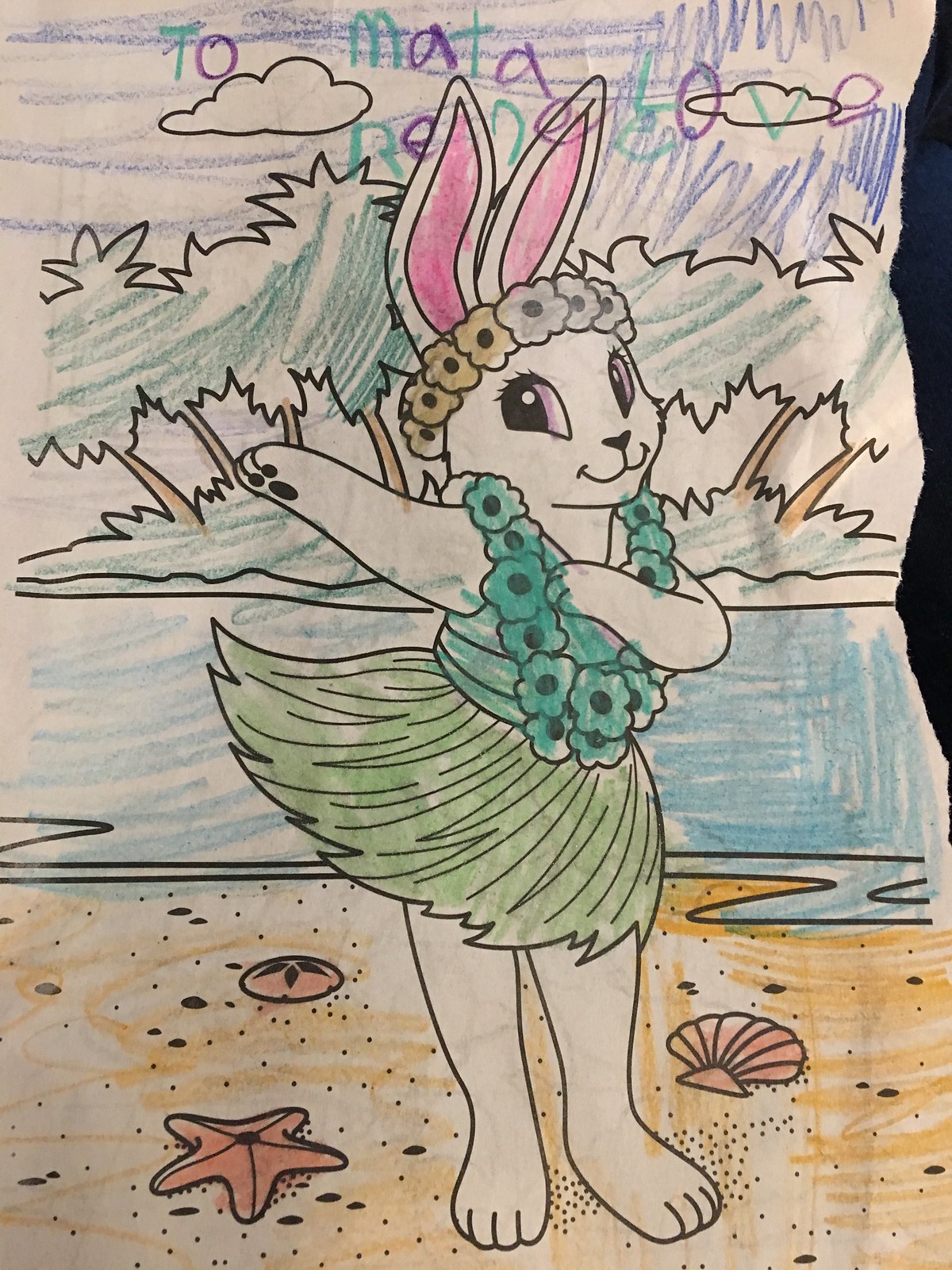In this vibrant image from a children's coloring book, a young artist has brought to life a whimsical scene featuring a humanoid rabbit. Colored enthusiastically outside the lines, the rabbit stands upright, reminiscent of a hula dancer, with one arm raised and the other resting near its chest. Adorned with a lei and shirt, both shaded a bold blue, the rabbit exudes a festive spirit further accentuated by a green grass skirt. A decorative floral headdress crowns its head, adding a touch of tropical elegance. The backdrop of the image sets the scene on a serene beach, scattered with seashells and framed by gentle waves. Behind the water, a lush island with towering trees completes this charming, lively seaside tableau.